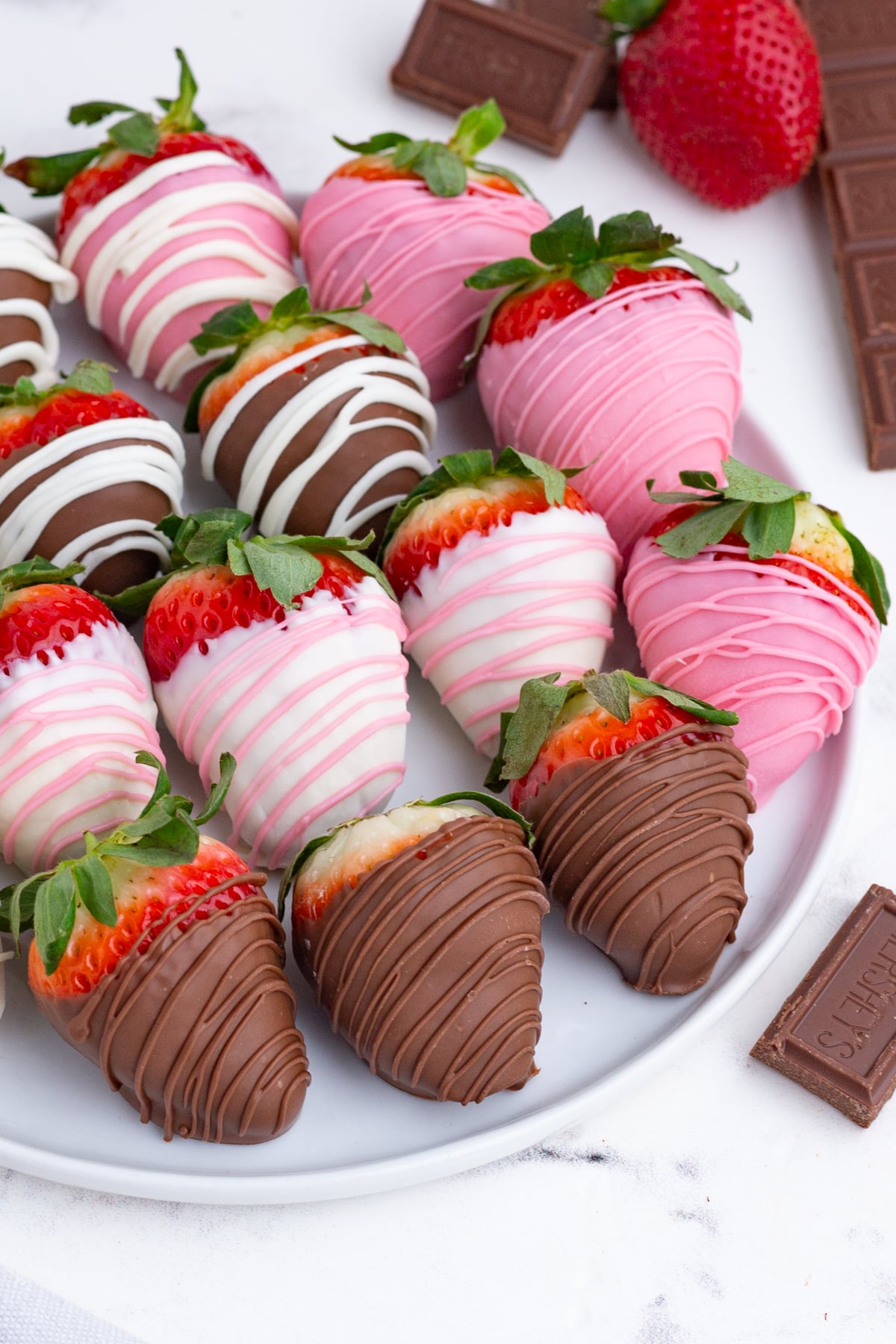In this detailed photograph, a white round plate elegantly displays about a dozen chocolate-covered strawberries, each adorned with various decorative patterns. The plate rests on a white marble countertop speckled with black, enhancing the visual appeal. The strawberries are intricately coated: some enveloped in milk chocolate with contrasting white stripes, others dipped in white chocolate with delicate pink stripes, and a few dressed in dark chocolate adorned with elegant white swirls. Towards the lower right of the countertop, a small Hershey’s chocolate square is visible, hinting at the chocolate's origin, with more chocolate bars and a whole, unadorned strawberry positioned in the upper right corner. This delightful assortment of treats, with its harmonious blend of colors and textures, promises a feast for the eyes and taste buds.